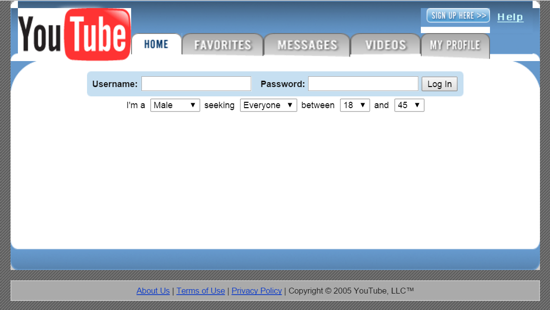This appears to be a screenshot from an early version of YouTube's homepage, around 2005. The browser window has a grey background with a bluish overlay. In the top left corner, the iconic YouTube logo is displayed, with "Y-O-U" in black and "tube" in white over a red rectangle shaped like a TV screen. To the right of the logo, the page features a series of tabs: the current tab "Home" in blue, and additional tabs "Favorites," "Messages," "Videos," and "My Profile" in grey. 

The main section appears to function as a login page, with fields to input a username and password. Below these fields, users could select demographic details from dropdown menus— "I am a male, seeking everyone between 18 and 45." This suggests that the platform had some social networking or matchmaking functionality at that time. 

In the top right corner, there is a prominent blue button labeled "Sign Up Here," next to a "Help" button. At the bottom of the screenshot, blue links indicate navigation options for "About Us," "Terms of Use," and "Privacy Policy," with "Copyright 2005, YouTube LLC, TM" written in grey beside them. This image offers a nostalgic glimpse into YouTube's interface and design from its early days.